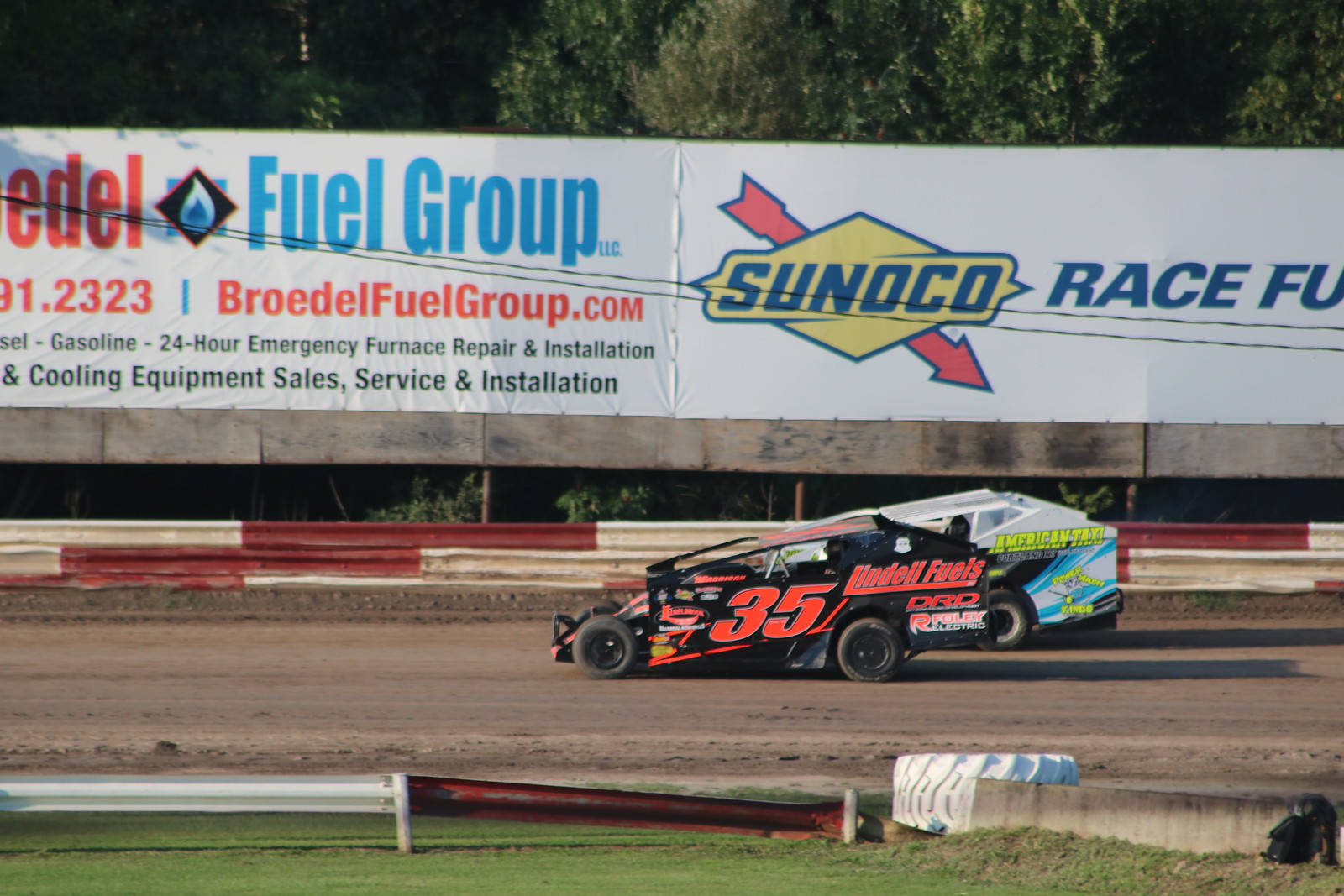In this image, we observe a vibrant racetrack scene dominated by two prominently featured rally cars in the center. The black car, marked with the neon pink number "35" and adorned with "Lindell Fuels" and "DRD" advertisements, is positioned closer to the camera. Overlapping slightly with this car is a gray vehicle detailed with neon green "American Taxi" signage. The dirt track they race on is bordered by a red and white metal guardrail, adding a sense of dynamic directionality that is reinforced by shadows cast to the right, suggesting light from the left.

In the foreground, patches of grass precede the track area while various structures such as a protective big white tire and concrete blocks create a safety buffer. Behind the guardrail, a large white billboard showcases multiple advertisements. Notably, this includes "Fuel Group" in blue letters, alongside "PROEDEL" in red. Detailed inscriptions mention services like gasoline, 24-hour emergency furnace repair, and cooling equipment service and installation, with a Sunoco label featuring prominently. The Sunoco logo, a yellow diamond with a red arrow and blue letters, partially reads "R-A-C-A" and "F-U," hinting at the word "race" and possibly "fuel," respectively.

In the background, a wooden fence is visible, beyond which tall trees blend harmoniously with the diverse color palette comprising green, gray, red, orange, yellow, blue, and tan. This outdoor scene is likely set in the middle of the day, providing a clear and lively depiction of a bustling race event.